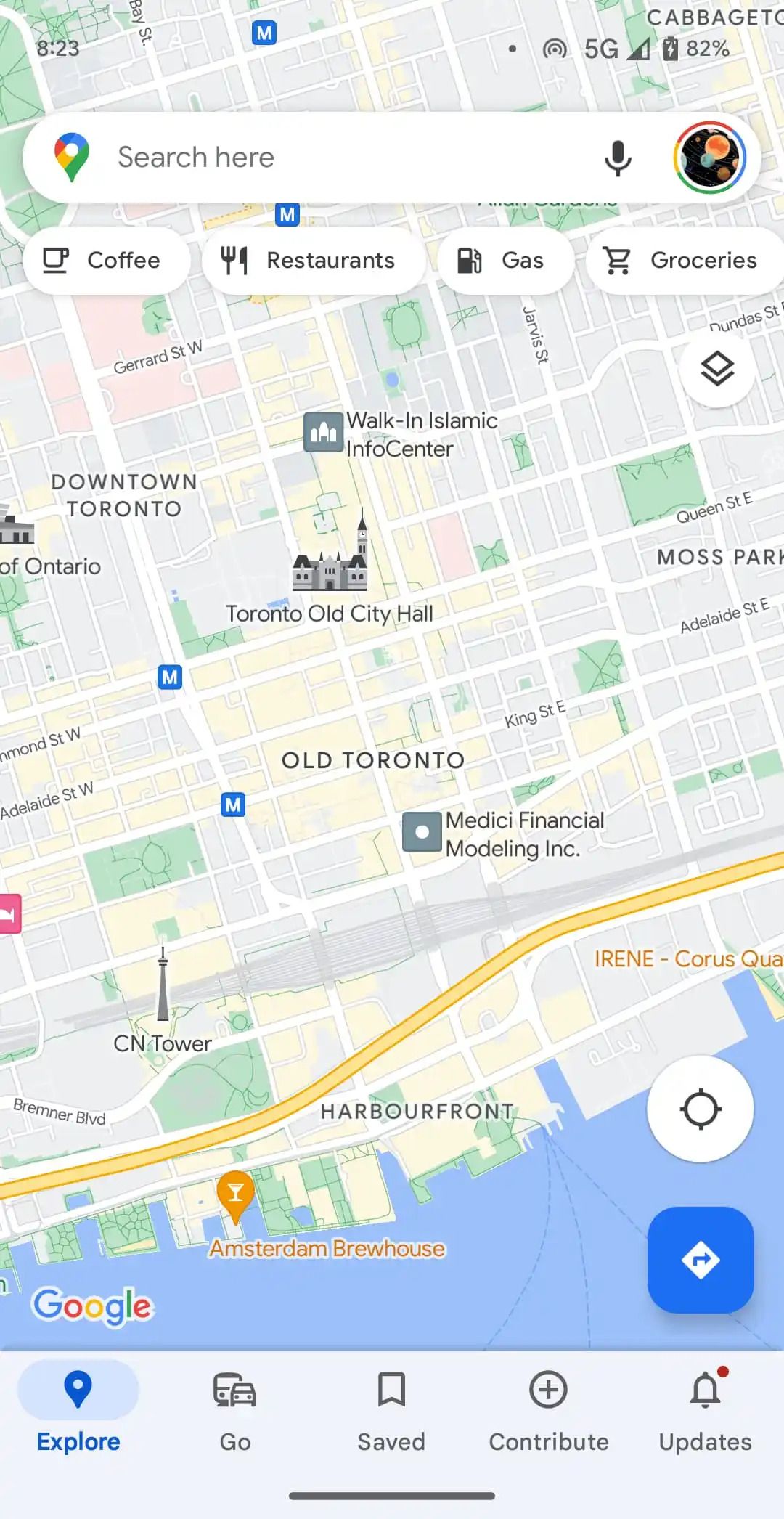The screenshot on the phone displays a detailed map of downtown Toronto. Prominently centered on the map is "Old Toronto," with "Toronto Old City Hall" positioned just above it, accompanied by a small icon depicting an older building. To the upper left, "Downtown Toronto" is labeled with another building icon next to the text "Walk-In Islamic Info Center." 

Towards the right of the screen, the label "Moss PAR" appears, possibly indicating Moss Park, situated near Queen Street and Adelaide Street. Moving south from "Old Toronto," "Medici Financial Modeling Incorporated" is noted, and to its left is the iconic "CN Tower." Further south and slightly to the right, "Harborfront" borders a waterway. A pinpoint below this indicates the "Amsterdam Brewhouse" restaurant.

Adjacent to the left near the bottom, the colorful Google logo is visible. Slightly north of "Harborfront," an obscured label reads "Irene Chorus" before running off the screen.

Additional details include the time at the top reading 8:23, a 5G icon, and battery status showing 82%. Below is a search bar with the prompt "Search here," accompanied by a Google-colored pin icon.

On the right side of the screen, there's a circular icon with an unclear image. Below it are four ovals, each representing different categories: "Coffee" with a coffee cup symbol, "Restaurant" with utensils, "Gas" with a gas pump, and "Groceries" with a grocery cart.

At the bottom, there are five navigation symbols, with "Explore" currently highlighted. The other options are "Go," "Saved," "Contribute," and "Updates."